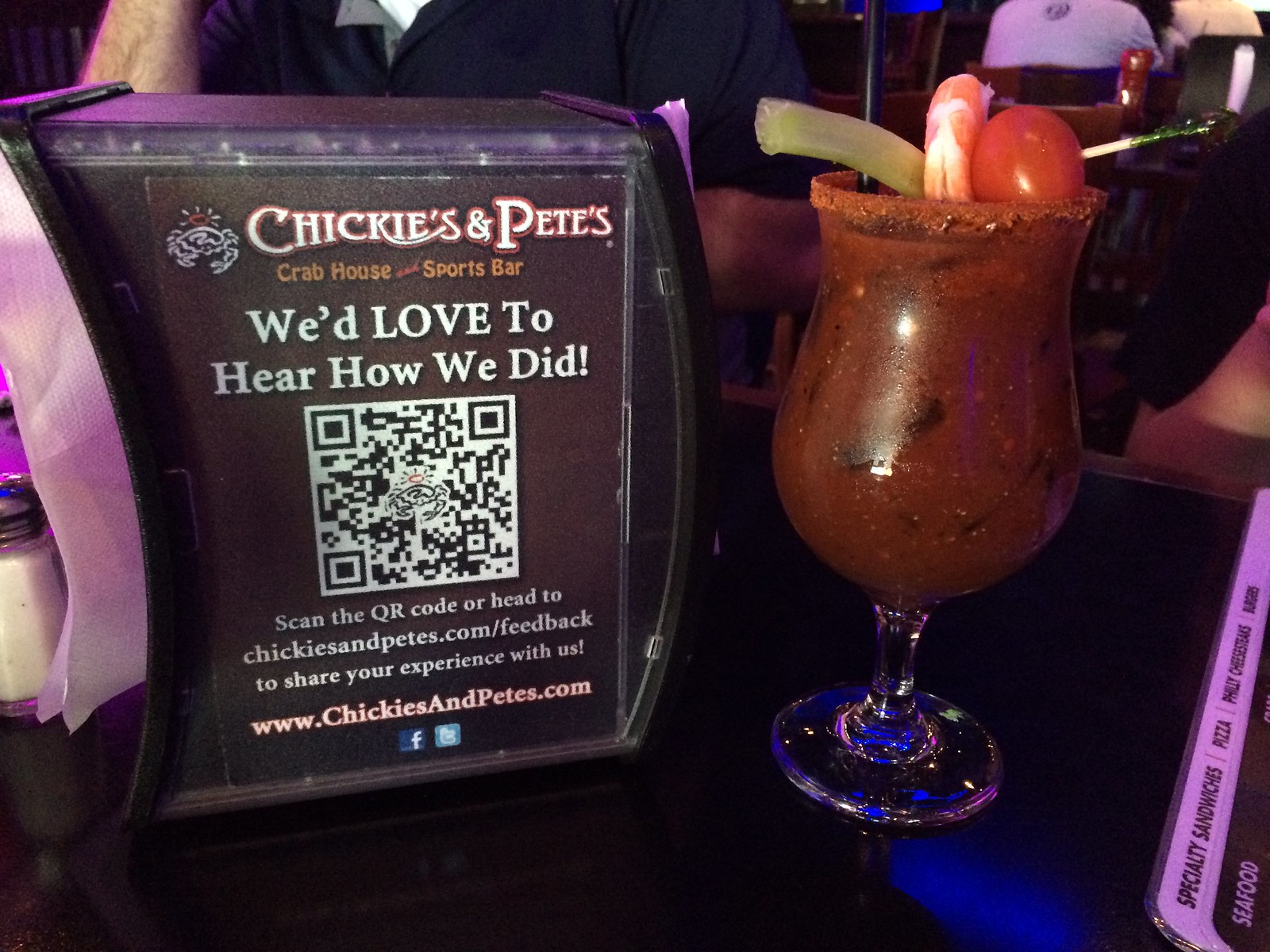The image depicts a dark, reflective table at a restaurant, adorned with a clear-stemmed glass filled with a brick-red liquid, likely a Bloody Mary. The drink is lavishly garnished with a piece of celery, a cherry tomato skewered on a green-tipped toothpick, and a shrimp, with a black straw emerging from the top. To the left of the drink, there is a purple napkin dispenser bearing white and orange lettering that reads "Chickies and Pete's Crab House and Sports Bar," along with a message inviting feedback via a QR code or their website, chickiesandpetes.com. The dispenser also features Facebook and Twitter icons. In the background, glimpses of other patrons and chairs provide a lively restaurant ambiance.